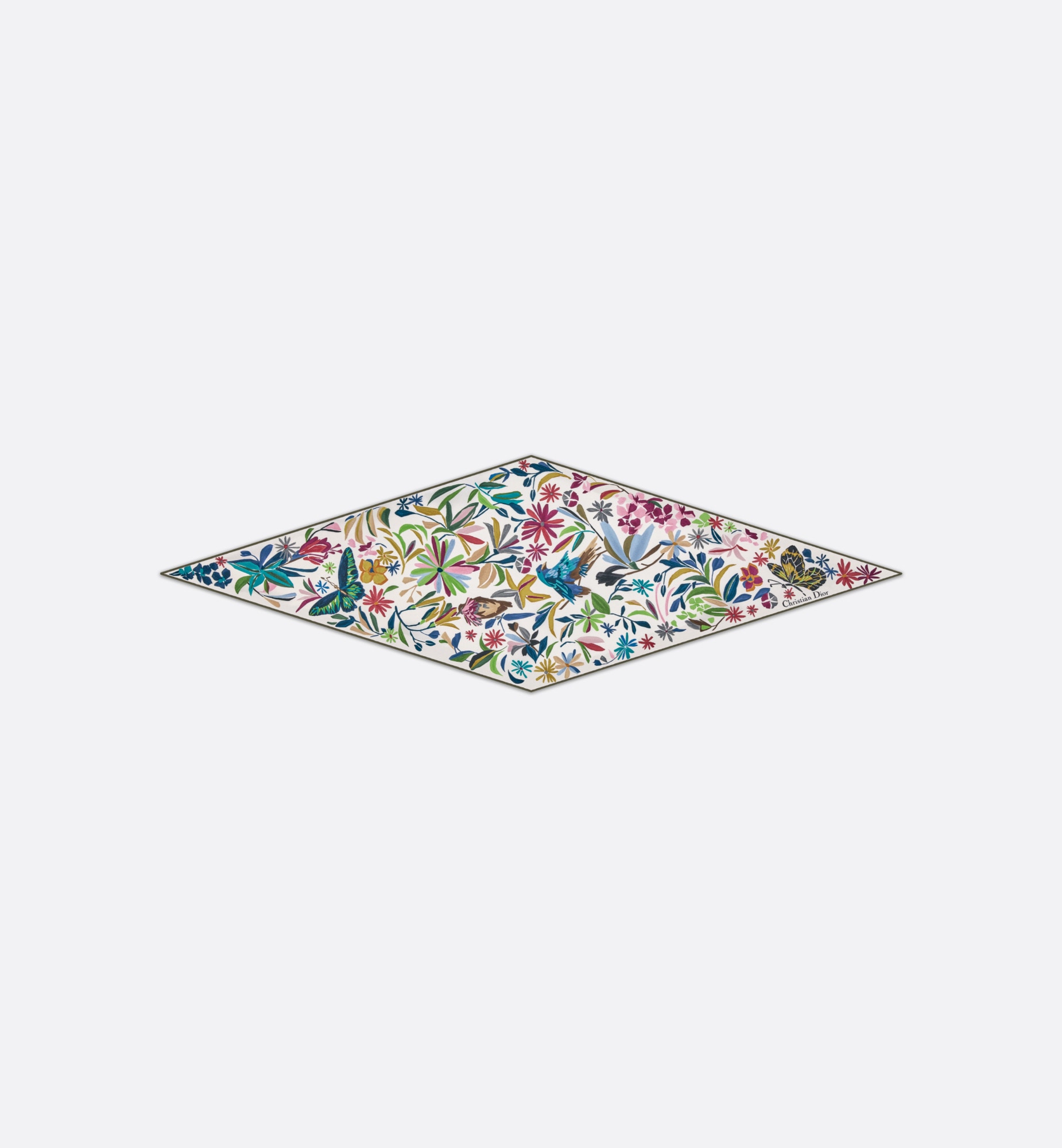The image features a centrally positioned diamond shape set against an all-white background. The diamond, oriented horizontally with its longer points extending sideways, serves as a canvas filled with an array of vibrant nature-inspired elements. Within the diamond, an intricate and colorful assortment of flowers, butterflies, dragonflies, birds, vines, and leaves creates a busy and visually engaging pattern. The primary colors within this nature collage include vivid greens, blues, and reds, with additional touches of yellows, pinks, and browns. Despite its simplicity, the diamond's contents are highly detailed, with dark black accents on butterfly wings adding depth. Although the diamond occupies only about a fifth to a quarter of the entire image, it stands out as an artsy and meticulously crafted focal point, embodying a rich array of colors and intricate floral motifs.